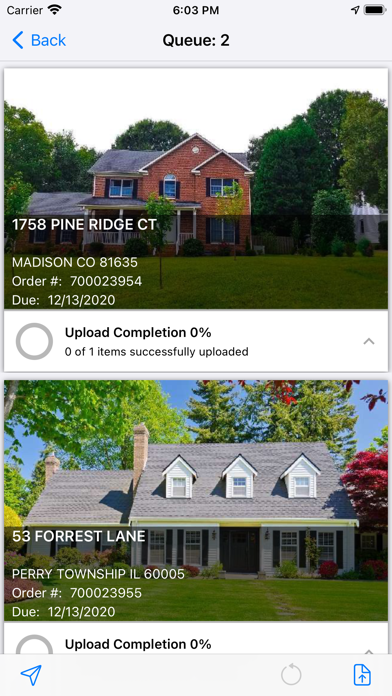This image appears to be a screenshot from a cell phone, potentially displaying a work order or task management system. In the upper left corner of the screen, the word "carrier" is displayed, indicating the network provider. The current time is shown in the center as 6:03 p.m., with a full battery icon in black located on the far right.

Below these indicators, there is a blue arrow pointing left accompanied by the word "back." Next to this, "QUEUE: 2" is indicated, suggesting two items in a queue.

The main body of the image features two properties listed for review:

1. The first property is a two-story brick Colonial house with a large front yard and green trees in the background. The address provided is 1758 Pine Ridge Court, Madison CO 81635. This entry includes an order number, 7000-23954, and a due date of December 13, 2020. Below this information, the status "Upload Completion 0%, zero of one items successfully uploaded" is shown.

2. The second property depicted is a Cape Cod-style house featuring two distinct chimney areas, a gray roof, dark blue shutters, and a well-maintained green lawn with trees in shades of red and green. The address for this house is 53 Forest Lane, Perry Township, IL 60005. It also includes an order number, 7000-23955, and a due date of December 13, 2020.